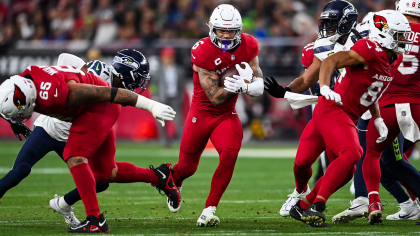A football player, clad in an all-red uniform, is captured mid-sprint while tightly clutching a football. His teammates, also in red, form a protective barrier around him, effectively blocking the opposing team. Although the player's jersey number is obscured, a faint number six appears to be visible on his shoulder. His muscular arms, adorned with intricate black tattoos, are strategically positioned to securely hold the ball. The player's white helmet adds a contrasting touch to his ensemble.

In the foreground, two opponents are visible. On the right side, a player in a black helmet and white jersey is being forcefully blocked by three red-clad teammates. On the left, another opponent, dressed in black and white with matching black pants, is dangerously close to tackling the ball carrier. His intense focus is evident as he zeroes in on his target.

Behind this intense action, a blurry sea of enthusiastic fans is visible, their cheers adding energy to the dramatic scene.